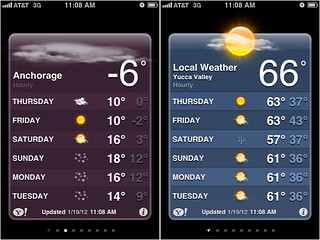The image displays a weather application interface with an assortment of detailed information. 

At the top of the screen, the status indicators show full signal strength on AT&T 3G at 11 AM with an almost full battery. The central part of the screen is predominantly purple and indicates that the location is Anchorage. The interface presents an hourly weather summary, showcasing a temperature of -6 degrees.

Here's the detailed weather forecast for Anchorage:
- **Thursday:** Cloudy, with a high of 10 degrees and a low of 7 degrees.
- **Friday:** Sunny, with a high of 10 degrees and a low of -2 degrees.
- **Saturday:** A high of 16 degrees and a low of 0 degrees.
- **Sunday:** A high of 2 degrees and a low of 12 degrees.
- **Monday:** A high of 16 degrees and a low of 12 degrees.
- **Tuesday:** A high of 14 degrees and a low of 10 degrees.

The data appears to be updated by Yahoo, with the timestamp showing as 1/19/12 at 11 AM. A circle icon labeled "I" also appears on the screen. Background information indicates the repetition of the word "time" multiple times.

Additional weather information is provided for Yucca Valley under the "local weather" category, showcasing mainly sunny and cloudy conditions.
Here’s the detailed forecast for Yucca Valley:
- **Thursday:** 66 degrees
- **Friday:** High of 63 degrees and low of 37 degrees
- **Saturday:** High of 63 degrees and low of 43 degrees
- **Sunday:** High of 57 degrees and low of 37 degrees
- **Monday:** Sunny, with a high of 61 degrees and a low of 36 degrees
- **Tuesday:** Sunny, with a high of 61 degrees and a low of 36 degrees

The Yucca Valley data also appears to be updated by Yahoo at the same timestamp, 1/19/12 at 11 AM. The image background is black, providing a stark contrast against the colorful weather information.